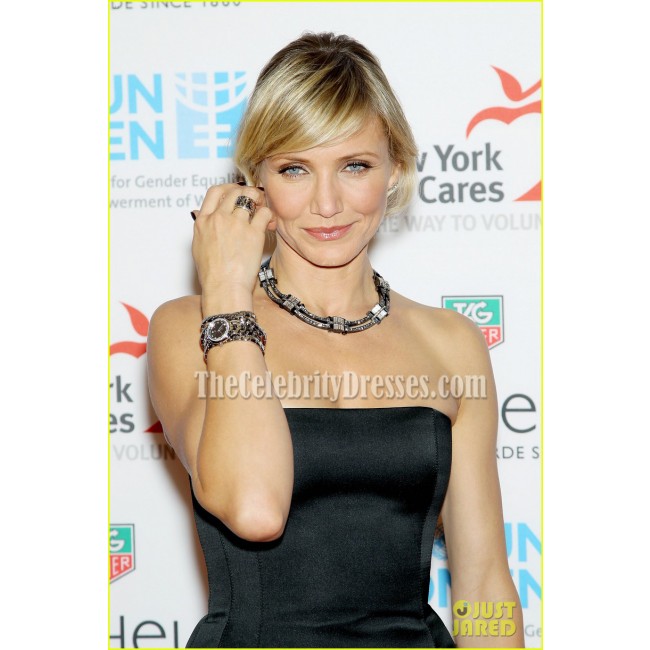In this photograph, Cameron Diaz is captured attending an event, standing confidently against a backdrop adorned with various logos promoting causes such as "New York Cares" and "Gender Equality". The backdrop suggests it is an award show or a promotional event. Cameron, who appears to be around 50 years old, exudes elegance in a sleeveless black dress that accentuates her statuesque figure. Her short blonde hair frames a radiant face as she smiles towards the photographers. She accessorizes with a striking, large metallic necklace, a prominent steel bracelet, and a matching watch, all adding a touch of flair to her outfit. A noticeable ring glistens on her finger. At the bottom right of the image, the URL "celebritydresses.com" is advertised, while the "Just Jared" watermark is also present. The image is primarily focused on her upper half, capturing her poised demeanor and chic style.